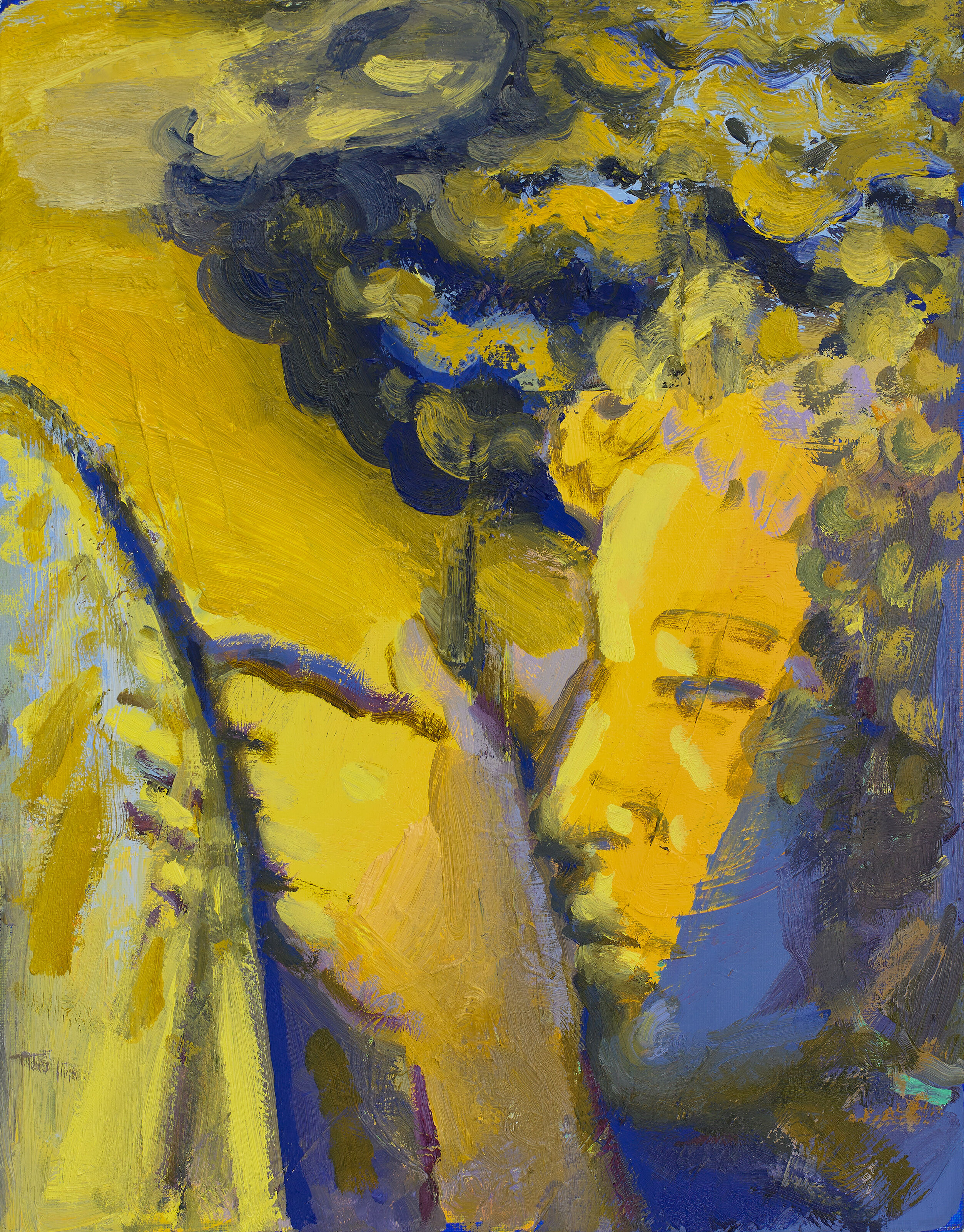The image is a vibrant oil painting featuring a side profile of a person's face rendered in shades of yellow, blue, and brown, with black highlights. The face is predominantly dark yellow with blue shadows emphasizing the contours, and bright yellow highlights reflecting light on the forehead and the front of the nose. The person's eyes and mouth are closed, conveying a serene expression. The left hand is raised in front of the lips and nose, suggesting a contemplative gesture. The hair is a blend of black, blue, and yellow tones, accentuating its texture. Surrounding the figure, the background consists of dark blues and yellows in wave-like patterns, adding depth and movement to the composition. The rectangular canvas captures the reflective light on various surfaces, hinting at a well-lit setting. Notably, an oval shape in front of the hand and face suggests the person is looking into a mirror, enhancing the introspective theme of the artwork.